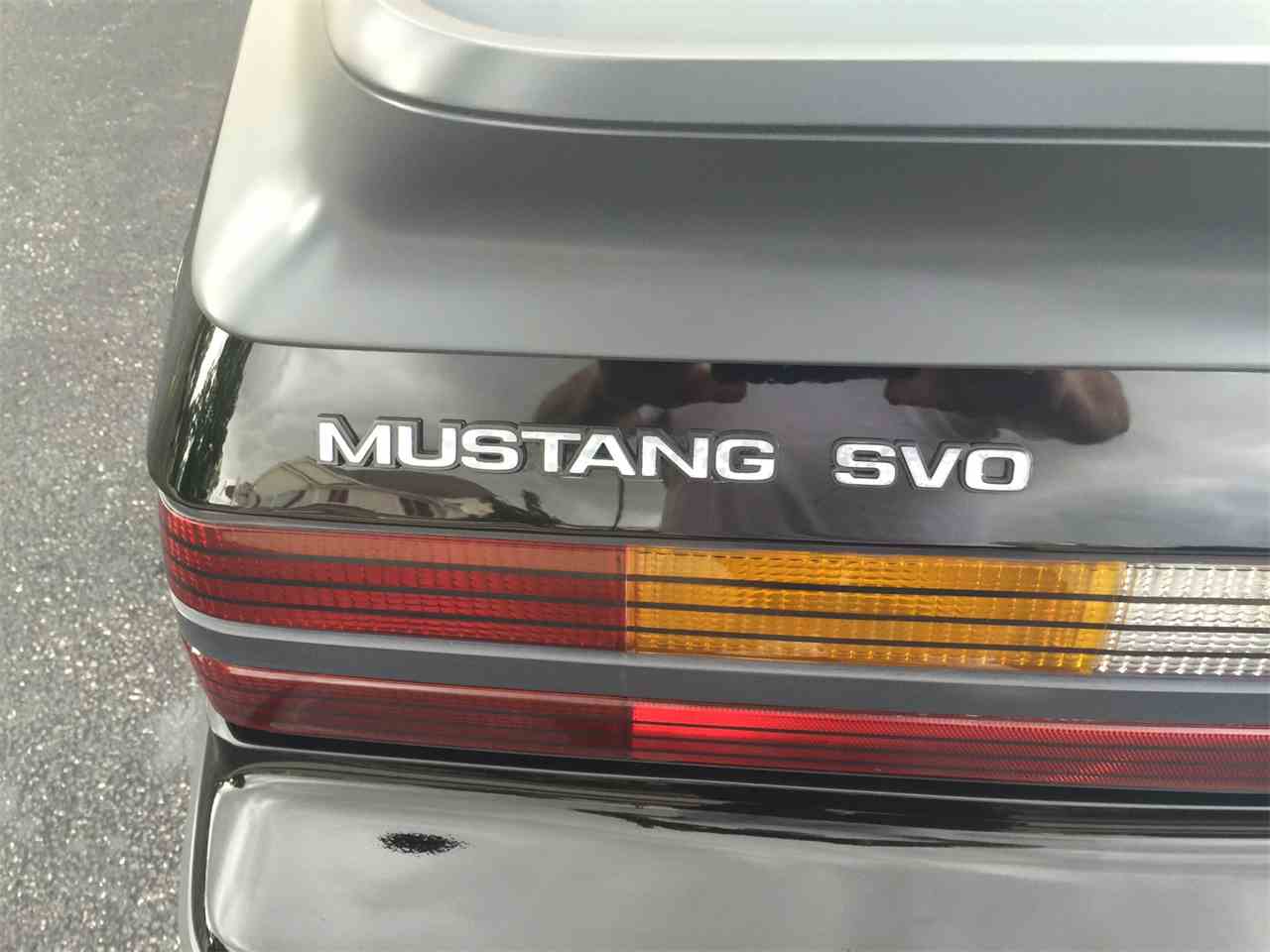The image captures a close-up view of the back left-hand corner of a shiny silver Mustang SVO, parked on light gray asphalt, possibly in a parking lot or on a street. Reflective black paneling on the car prominently displays the text "Mustang SVO" in white letters. Within this panel, you can discern the reflection of a person, likely the photographer, wearing a white or light pink shirt with hands positioned on either side of the camera. Also reflected in the glossy surface is the faint image of a house. Below the text, the car's taillights are visible, featuring a sequence of colors: a red rectangle followed by yellow and white segments, with additional red lights and a gray thin rectangular piece below. The car’s clean and shiny exterior is evident, indicating that it appears very new and well-maintained.